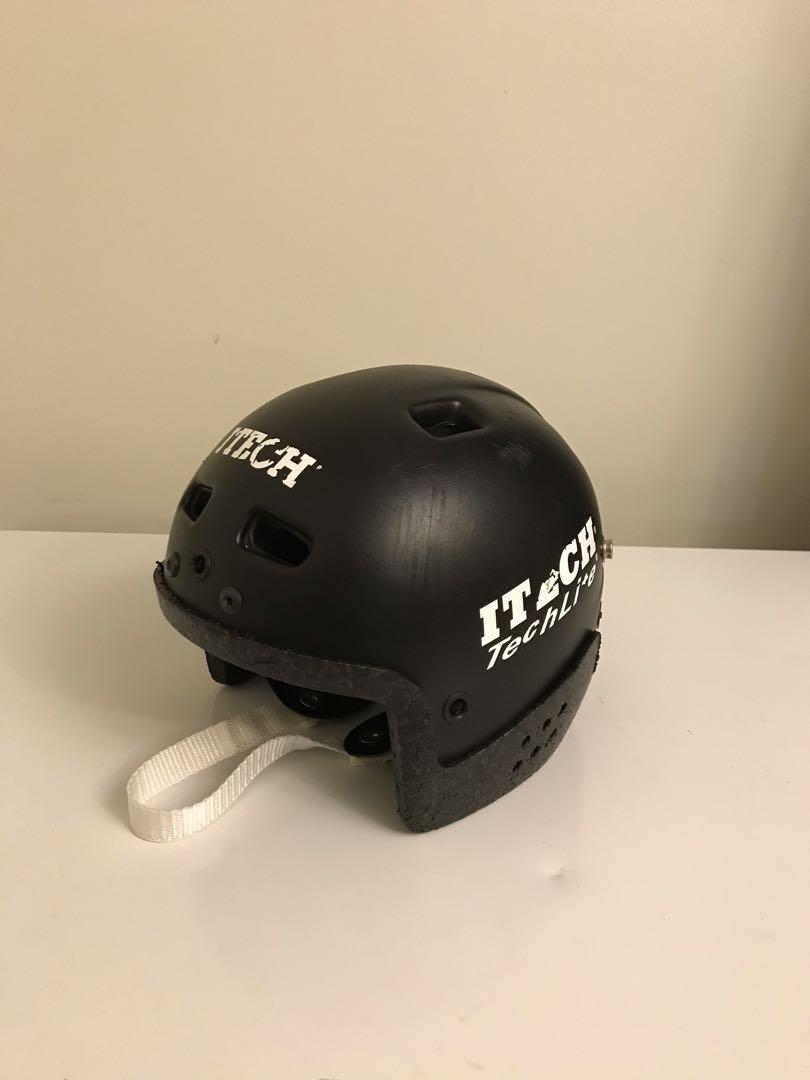The image displays a black sports helmet prominently placed on a white table against a white wall or beige background. The helmet, made of plastic, features a series of black square cutouts on the top and along the front for ventilation. On the helmet's surface, large white letters spell "Tech," though portions of the lettering are either cut off or slightly peeled, particularly making "IT" and "CH" visible on the right side of the helmet. Below these larger letters, the words "Tech Light" appear in thin white lettering. A white chin strap is also visible, resting on the table next to the helmet. The overall image is clear and well-lit, focusing solely on the helmet without any other objects in the frame.